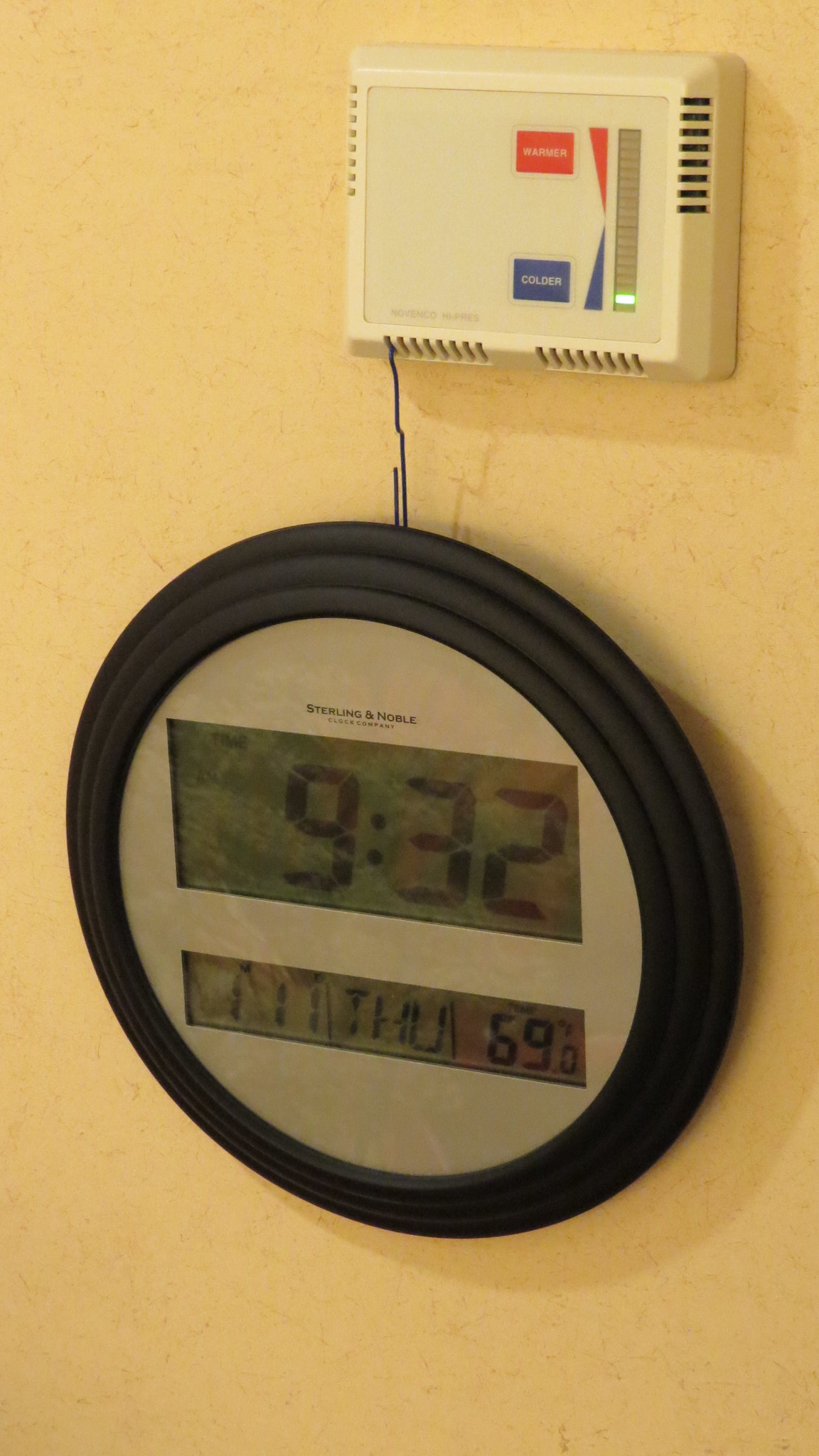This is an image featuring a round electronic device encapsulated in a black frame with two LED screens. The larger screen, positioned at the top, is horizontally oriented and displays "9:32" in bold black numerals against a lighter background. Below this time display is a second section exhibiting a series of numbers and separated by thin lines. It reads "THU," likely indicating Thursday. To the left of "THU" are three numeral ones (111), and to the right, the temperature is shown as "69 degrees."

The round device is suspended or hung using an unfolded paperclip, which is attached to a nearby thermostat situated about an inch above it. This thermostat has a horizontally oriented, rectangular shape with an electronic display bearing a green bar near the bottom. The bar is segmented and labeled with a blue box at the bottom marked "colder" and a red box at the top marked "warmer." This display includes long, narrow pyramid shapes that taper from a wider base to a narrow top, transitioning in color from red at the top to blue at the bottom.

All these elements are set against a yellow wall, accentuating the contrast between the device, its display information, and the background.